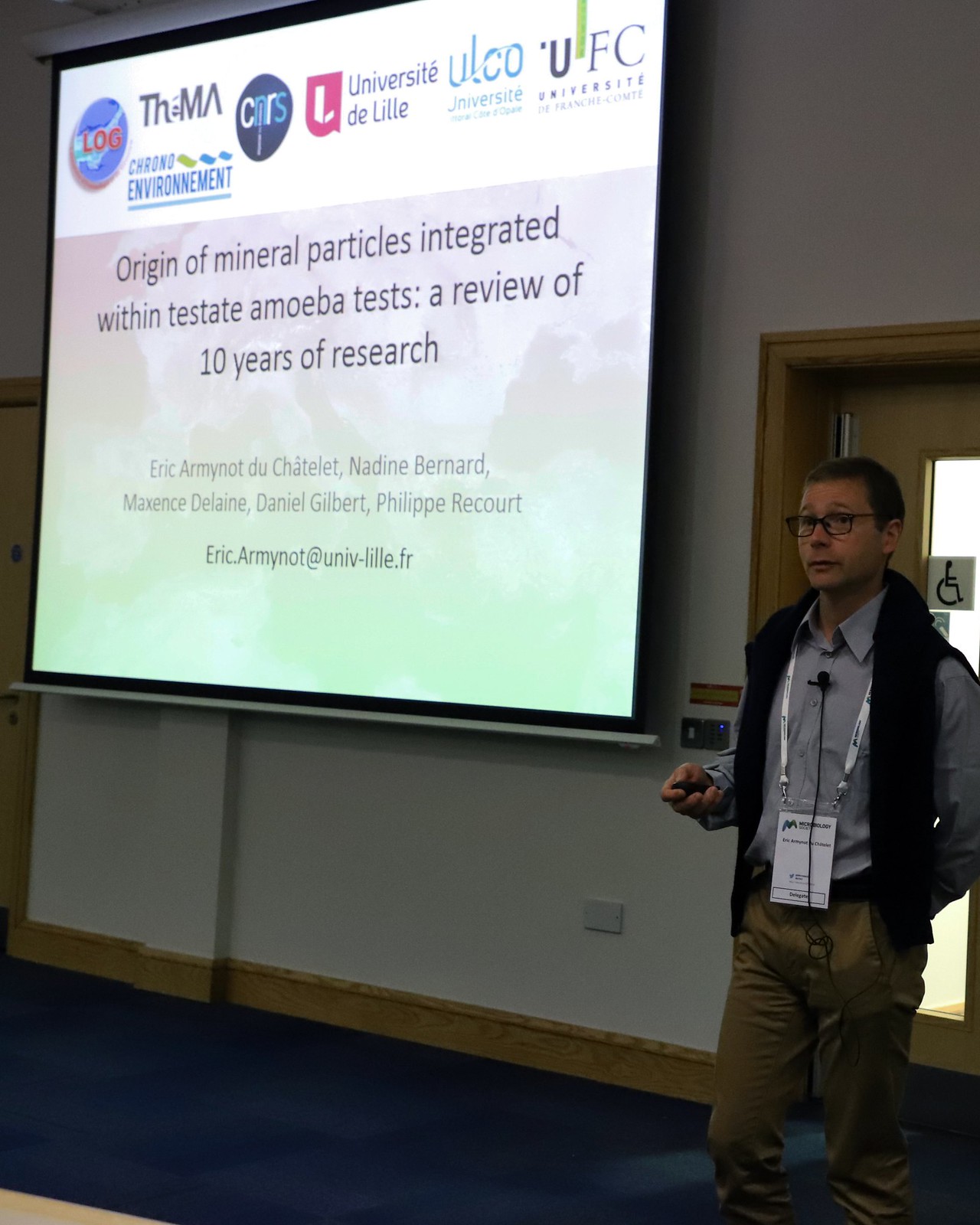In the image, a gentleman, approximately in his 40s, stands on the right side in what appears to be a college classroom, next to a door marked with a wheelchair logo, indicating accessibility. He is dressed in a black vest over a grayish-blue long-sleeved shirt, with brown pants, and he is wearing glasses. A laminated name badge hangs around his neck, a microphone is clipped to his shirt, and he holds a clicker in his hand as if about to advance the presentation on a large screen to his left.

The screen displays text which includes various academic institutions and research organizations: "LOG," "THMA," "Crono," "Environment," "CNRS," "University D Lille," "ULCO," and "UFC University." The central title of the presentation reads, "Origin of Mineral Particles Integrated Within Testate Amoeba Tests, a Review of 10 Years of Research." At the bottom, the names "Eric Armanot Du Chatelet," "Nadine Bernard," "Maxine Delane," "Daniel Gilbert," and "Philip Ricourt" are listed as contributors. The screen also shows a contact email: "eric.armanot@univ-lille.fr."

The combination of his attire, the microphone, and the detailed academic presentation suggests he is likely presenting his research at a conference or academic convention.